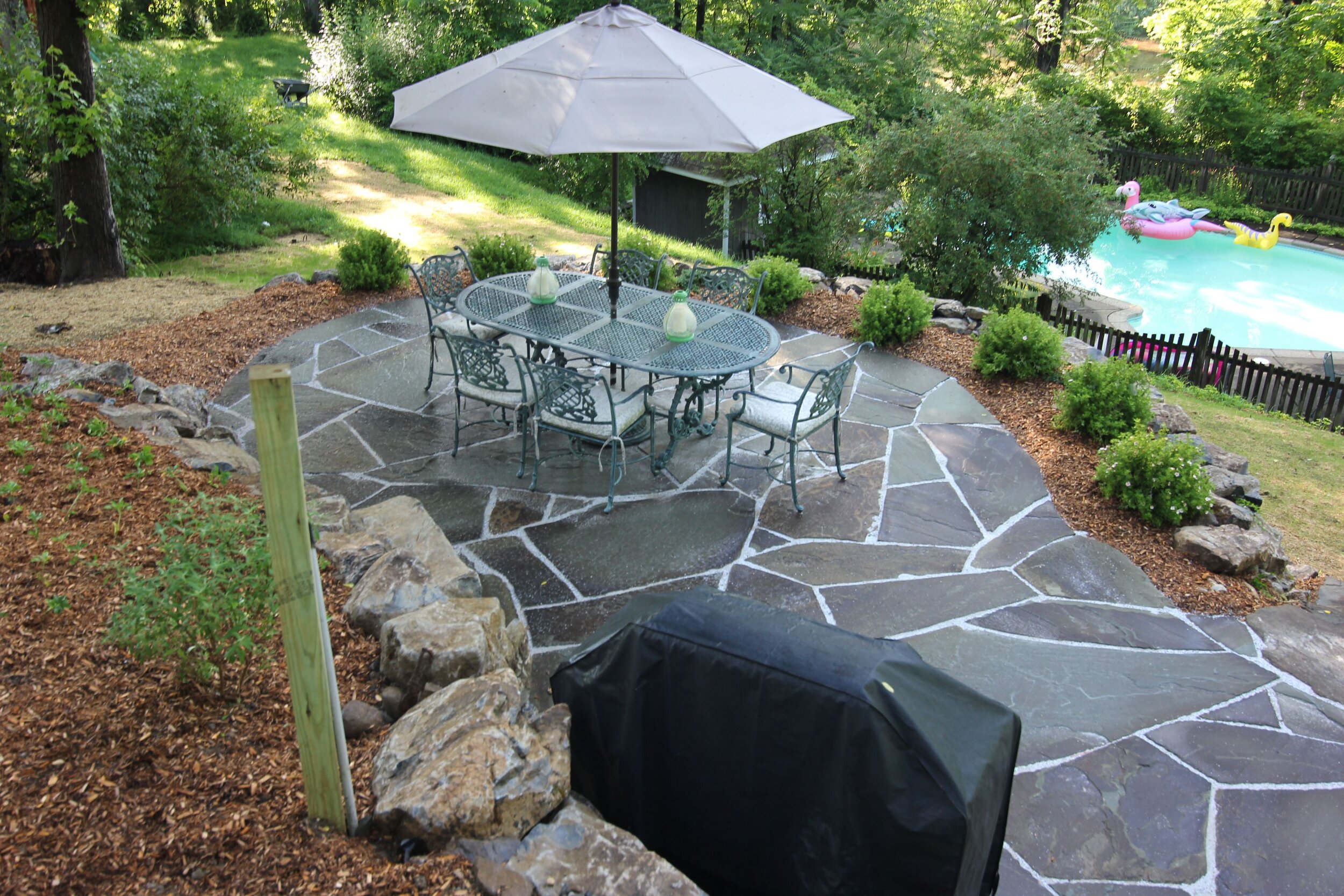This vibrant, full-color photograph captures a serene outdoor scene on a bright and pleasant day, likely in someone's backyard. The image is square, featuring lush greenery with verdant leaves framing the top. Sunlight filters through the canopy, illuminating parts of the foliage on both the left and right sides. 

Central to the composition, on the right side, is a swimming pool surrounded by a brown picket fence. The pool hosts playful inflatables, including a pink flamingo, a yellow dinosaur, and possibly a blue dolphin. Nestled within a forest-like lawn area, the pool radiates a sense of leisure and fun.

Elevated above the pool, a black stone patio is adorned with a black wrought iron table, six chairs, and a patio umbrella. Here, a barbecue grill covered in a black cover stands nearby. The table and chairs are set on an intricate surface of stone tiles in various sizes, situated on a gentle hill. Higher up, more terraced landscaping adds to the visual depth and greenery of the scene, with trees gracefully enveloping the entire area.